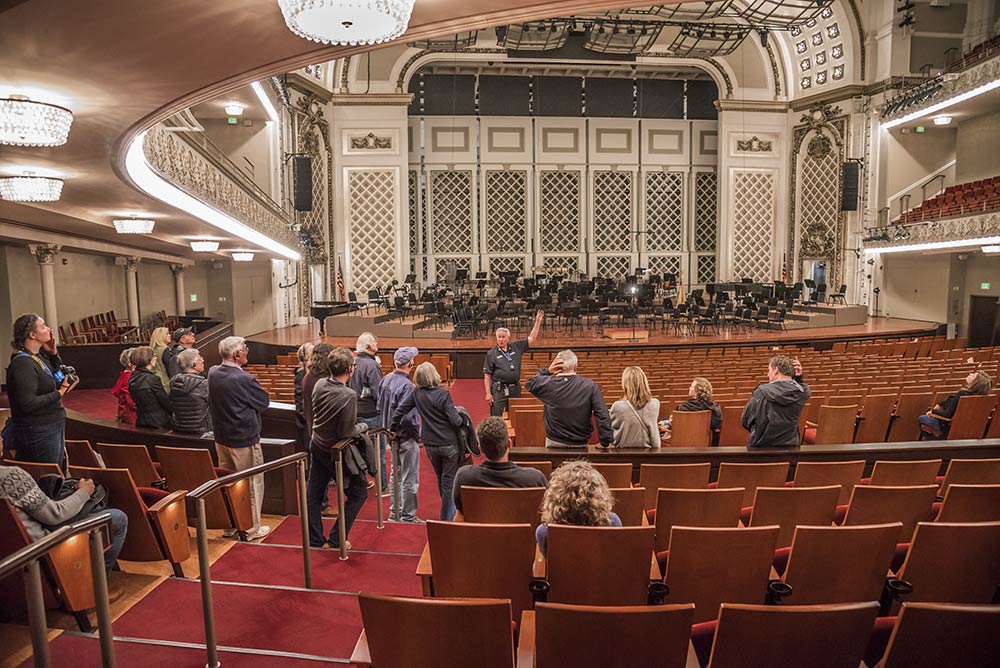The photograph captures an elegant and historic orchestra hall or auditorium, meticulously detailed and richly adorned. The scene is centered around a tour group, attentively guided by a man dressed in a black polo and pants. He stands on the left-side stairwell, arm raised, illustrating the grandeur of the hall to a mixed group of standing and possibly seated individuals. The guide’s gesture encompasses the entire space, drawing attention to its multiple seating sections: three on the ground floor, a balcony level above, and one more balcony tier at the top.

The orchestra stage itself is set with neat rows of black chairs and matching music stands, staged against a distinctive beige latticework backdrop composed of wooden crosshatch panels extending across the rear of the stage. The stage floor is a polished light wood, creating a distinguished contrast with the dark furnishings. 

The audience seating is cozy with mahogany-colored wooden chairs, red velvet-padded seats, and wooden armrests. The stairwells feature plush burgundy carpeting, complemented by practical handrails for added safety. The hall's sophisticated aesthetic is further enhanced by cream-colored walls and grand crystal chandeliers that exude old-world charm. This comprehensive description reveals the auditorium as a place of both beauty and history, vividly brought to life by the detailed observations of the tour guide.